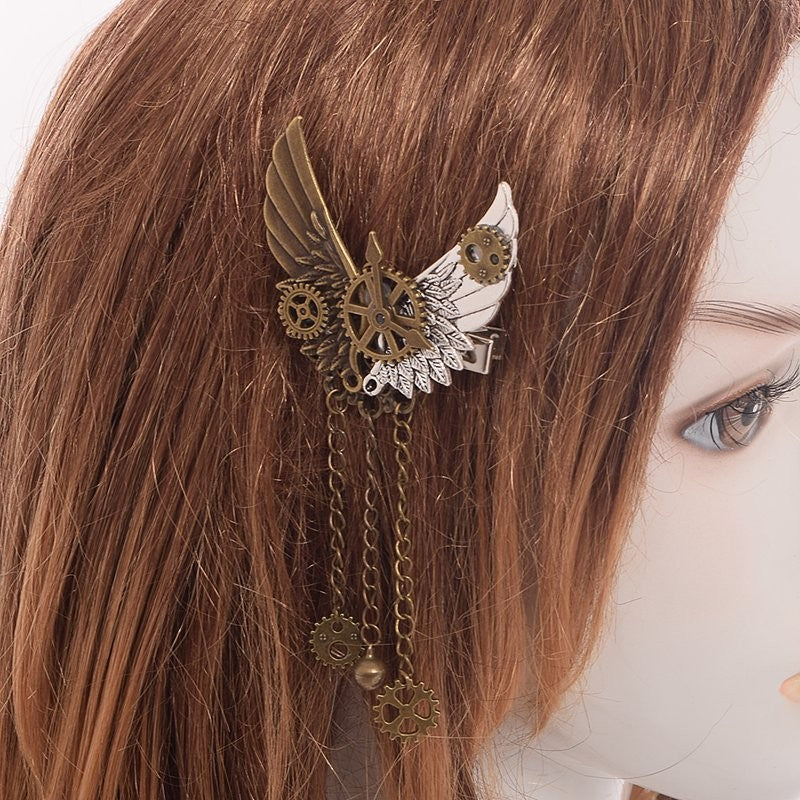This photograph features the head of a mannequin with long, straight, reddish-brown hair that cascades down across the side of its white, expressionless face. The focal point of the image is a detailed hair ornament clipped to the right side of the mannequin's hair. The elaborate pendant, resembling a steampunk design, includes two wings—one copper and one white—with intricate, stylized feathers. At the center of the pendant, a brass gear is decorated with clock hands extending outward. Three chains dangle from the wings, each contributing to the intricate design. The two outer chains end with small gears, while the middle chain culminates in a tiny copper sphere. This striking hair accessory, coupled with the mannequin's vividly colored hair, creates a visually compelling and detailed composition.